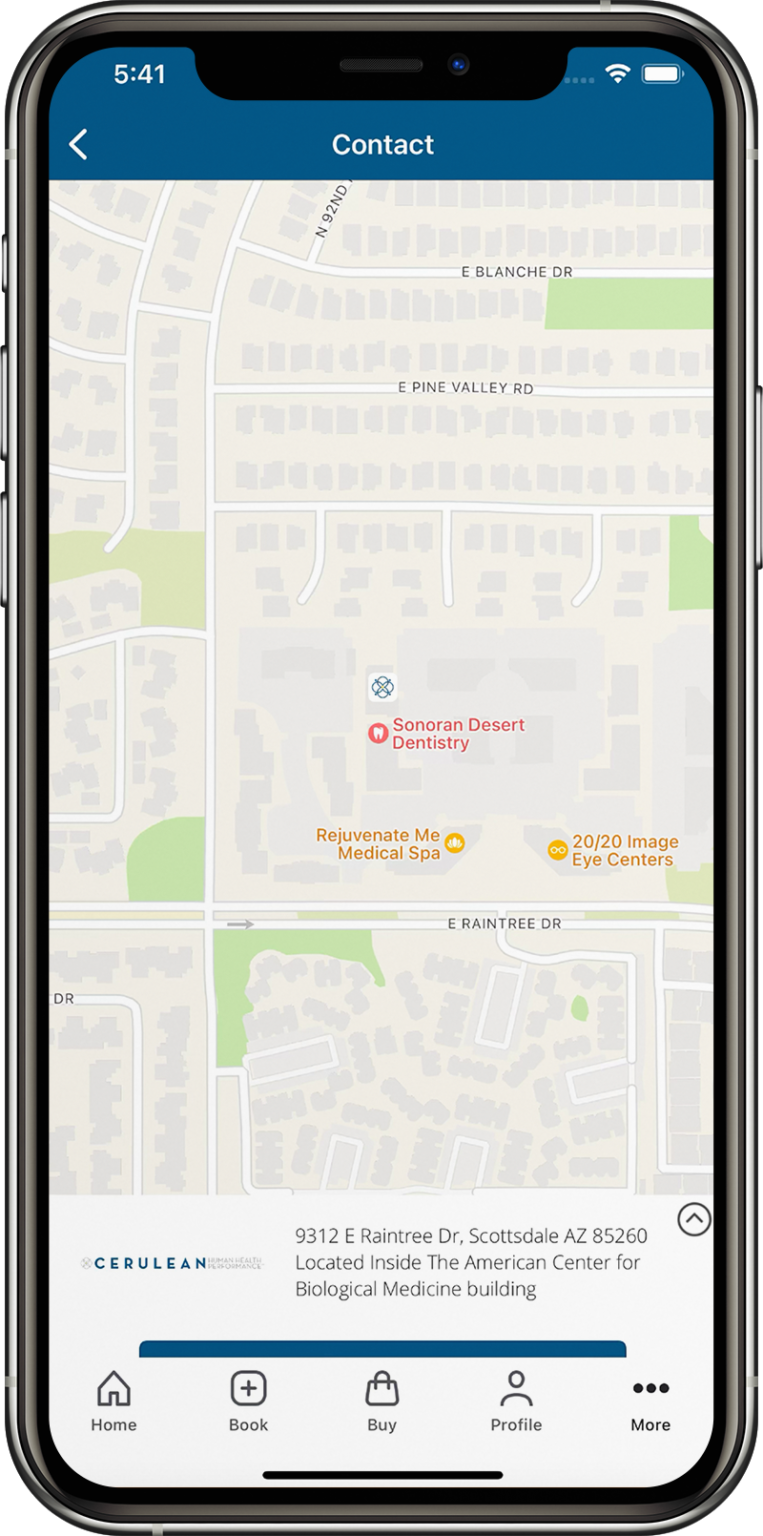A screenshot captures the entirety of a smartphone's front face, showing the familiar external buttons and sleek exterior edges typical of an Android device. At the top, you can see a sensor bar, speaker, and a camera lens. The device indicates it is 5:41, with a full battery and a strong internet connection. The screen displays an application, though its specific purpose is unclear. At the bottom of the screen, there is a navigation bar with options labeled "Home," "Book," "Buy," "Profile," and "More."

The primary content of the image focuses on contact information and a map highlighting streets and nearby businesses. Notable establishments include Sonoran Desert Dentistry, Rejuvenate Me Medical Spa, and 2020 Image Eye Centers. At the bottom of the screen, more detailed information is provided about a location named Cerulean, situated at 9312 East Raintree Drive, Scottsdale, AZ 85260, inside the American Center for Biological Medicine building. The image is straightforward, mainly featuring the discussed elements without additional distractions.